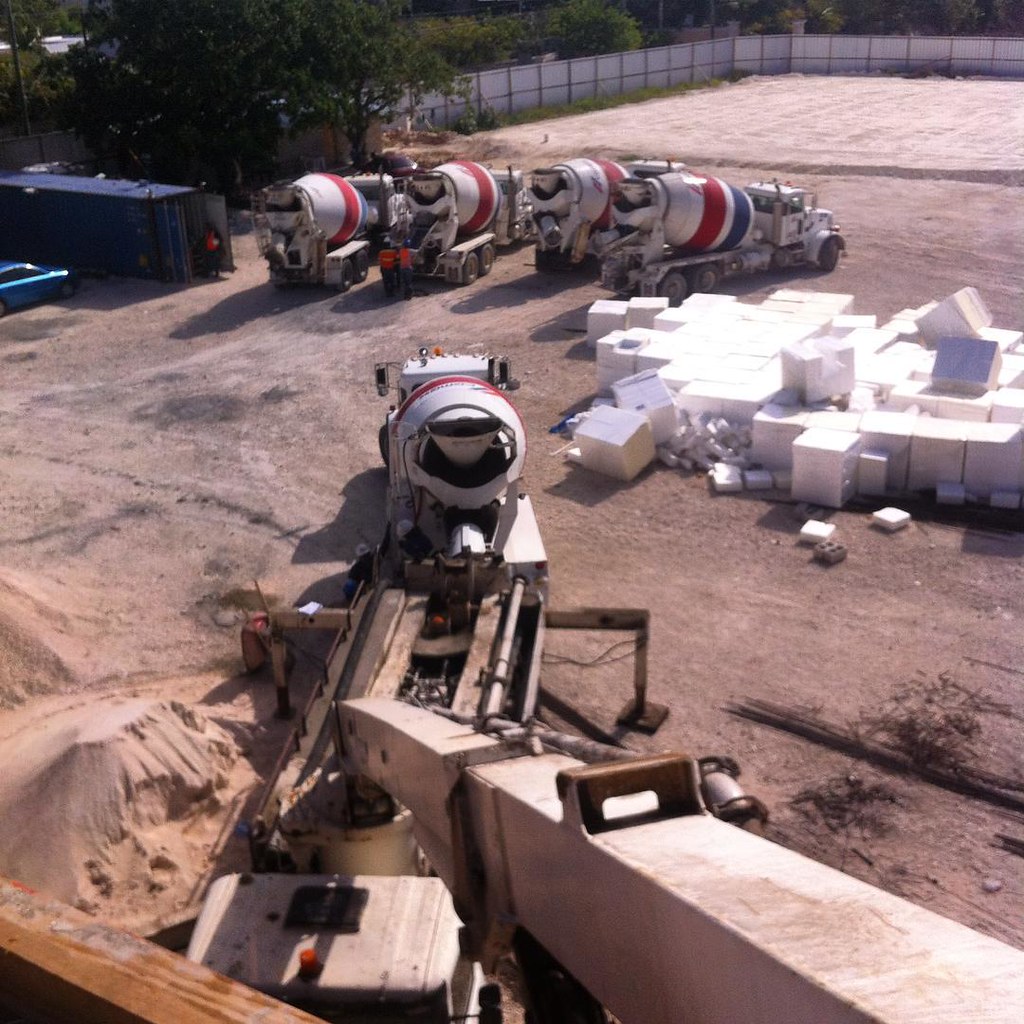The image depicts an expansive construction site viewed from an elevated perspective, possibly three or four stories up. The ground is predominantly dirt, and in the upper portion of the image, there are four cement trucks lined up in a row. Each truck features a distinct white barrel adorned with a large blue stripe near the cab, followed by a narrow white stripe and a broad red stripe. One of these trucks is positioned toward the back, appearing to be unloading cement via a rectangular apparatus into a platform or bed behind it. 

On the right-hand side of the image stand several large white cubical structures, which look like massive blocks of Styrofoam, all neatly arranged side-by-side. Adjacent to the left, there's a mound of sand, adding to the busy construction scene. Additionally, a blue trailer or shipping container with open doors is visible, and three people can be seen in the vicinity—all wearing red shirts. Two people stand behind one of the cement trucks, while another person is inside the doorway of the trailer. A white fence delineates the far background of the site, enclosing the area.